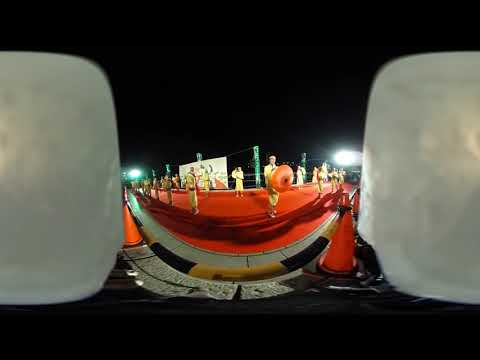The photograph captures a nighttime outdoor performance on a stage covered with an orange-red carpet. Despite the image's slight blur and distortion, perhaps due to a panoramic or fisheye lens effect, you can clearly see a group of people dressed in yellow uniforms. Some participants are holding traditional Chinese-style parasols in orange. The edges of the stage are lined with orange traffic cones, creating a boundary, and surrounding this stage is a black and yellow dashed curb. Shadows stretch across the carpeted stage, enhancing the nighttime atmosphere. In the background, there are green posts with a white sign attached by strings, adding to the intricate scene. Although there's a poster or framed artwork behind the performers, the text remains unreadable. The sky is completely black, emphasizing the outdoor nighttime setting.